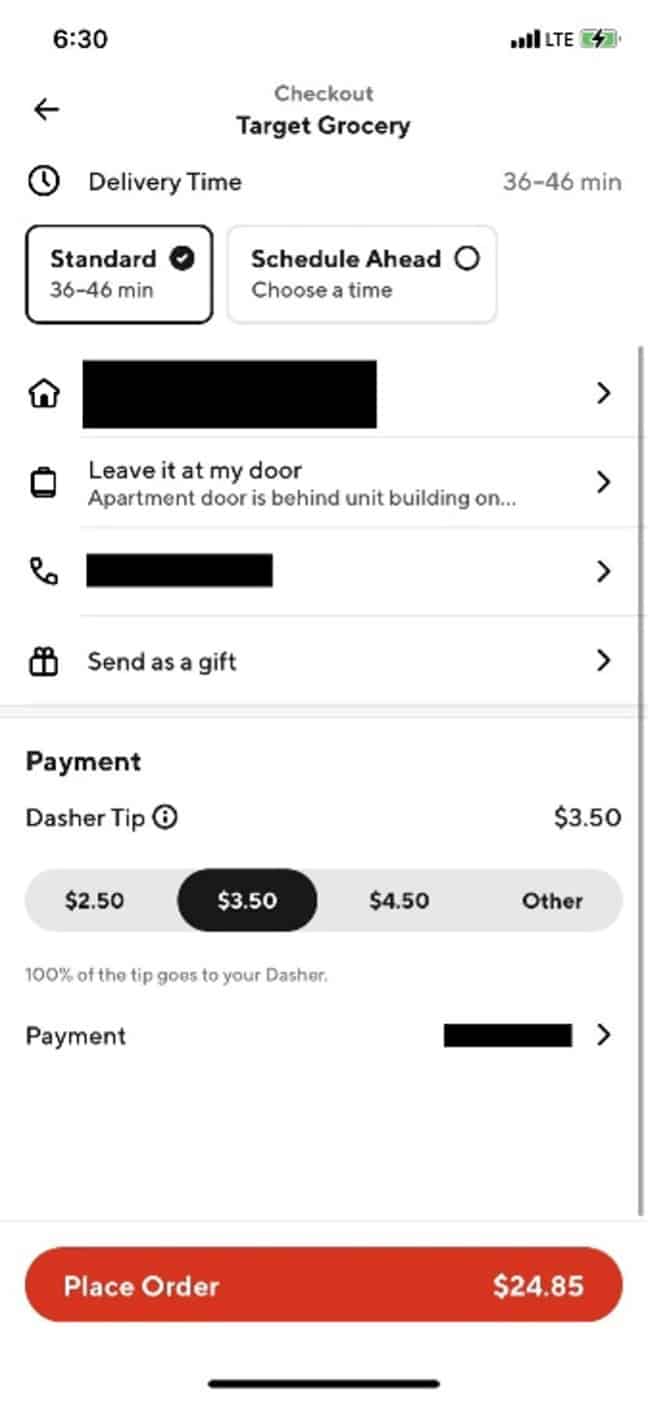This is a detailed screenshot of a cell phone displaying the checkout page from Target Grocery. The time, shown in the upper left-hand corner of the screen, reads 6:30. The central part of the screen features the title, "Checkout from Target Grocery," where "Checkout" is displayed in gray text, and "Target Grocery" is in black text beneath it. Directly below, on the left side, it shows the delivery timeframe as "36 to 46 minutes."

Two selection boxes appear below the delivery information. The first option, which is selected, is labeled "Standard: 36 to 46 minutes." The second, unselected option is "Schedule Ahead: Choose a time." An address, which has been redacted for privacy, appears beneath these options.

Further down, the text instructs to "Leave at my door," specifying that the "apartment door is behind unit building." The phone number for the order has also been redacted. Below this information, there is an option labeled "Send as a Gift."

At the bottom of the screenshot, the order total is displayed, amounting to $24.85.